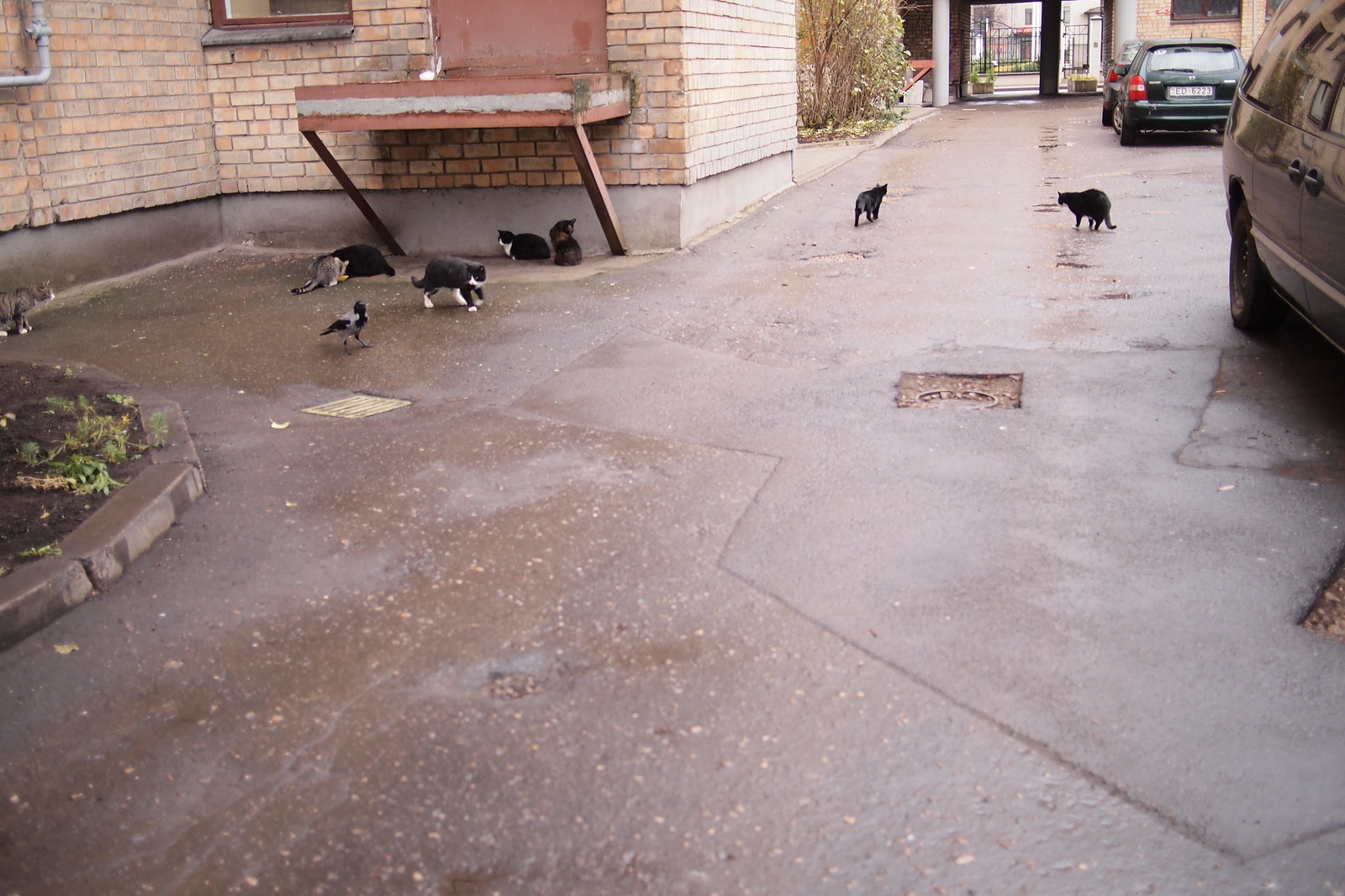In this image, we see a group of seven stray cats, primarily black with some having white paws and necks, gathered in what appears to be a wide, wet alley or parking area next to a brick building. The building features a reddish-orange to tan brick façade and a rusty wooden platform, which might be a disused loading dock supported by diagonal joists. Two gray cats are also present, and a pigeon or crow stands among them. Most of the cats are gathered beneath the platform, possibly seeking shelter from recent rain, while a few others are walking around. On the right side of the image, there are three parked vehicles, including a van and cars. The area is somewhat grim and not very colorful, featuring potholes and an overgrown weedy planter on the left. Towards the back of the scene, a black gate and some greenery are visible, adding to the urban, slightly desolate atmosphere.